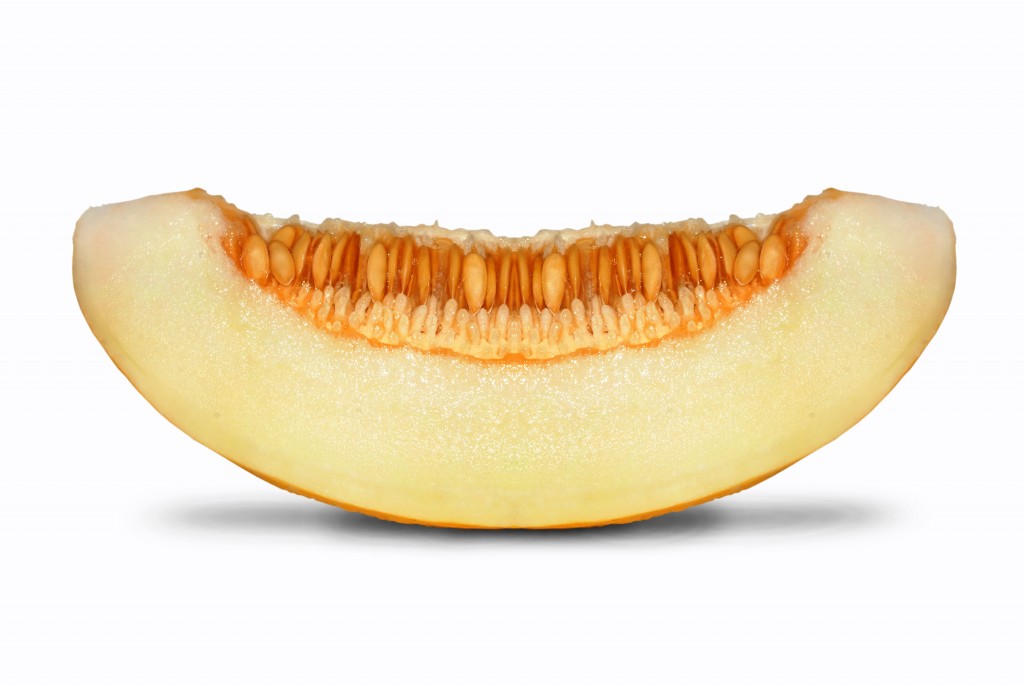This photograph features a single, curved slice of cantaloupe, prominently displayed against a stark white background that emphasizes its shape and colors. The cantaloupe slice forms an almost semicircle, with its light yellowish cream flesh showcasing a cluster of orange and cream-colored seeds arranged horizontally along its inner curve. The simplicity of the image, devoid of any text or additional elements, directs all attention to the cantaloupe. A subtle shadow beneath the slice adds depth to the image, creating a slight gray hue against the otherwise pristine background. This minimalist composition highlights the natural beauty and detailed texture of the cantaloupe and its seeds, making it suitable for a food website or a similar context where the focus is on the fruit itself.